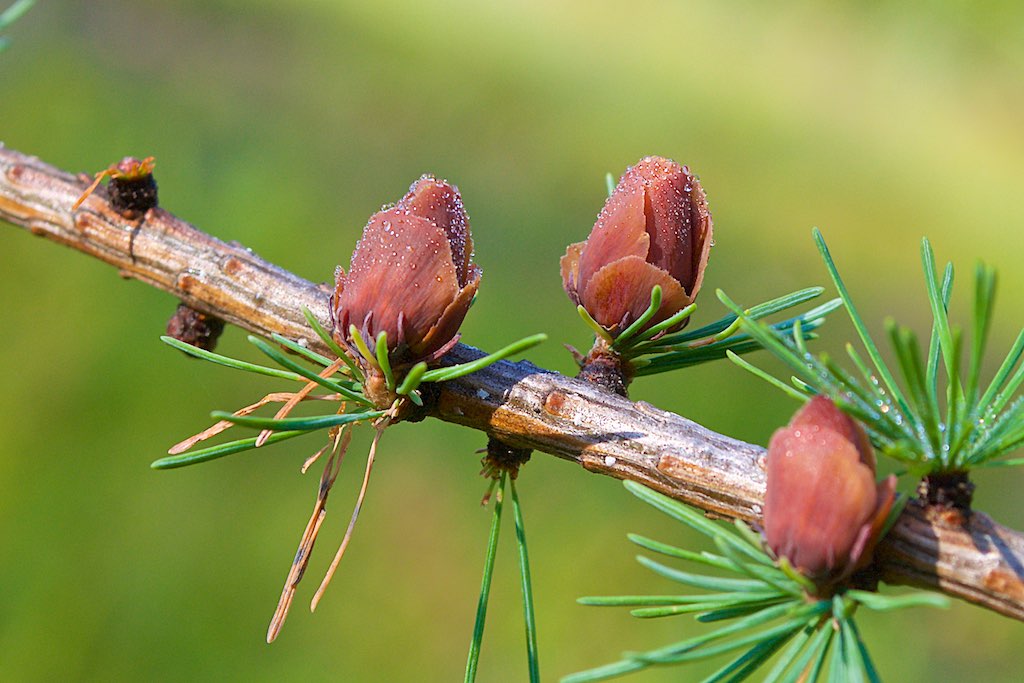In this detailed nature photograph, a thick, brown wood branch stretches across the frame, adorned with partially developed pine cones that resemble closed roses with their layered, brown appearance. There are three distinct pine cones, some encircled by clusters of green pine needles, while others have fewer surrounding needles. Emerging pine cones are also visible, indicating new growth. The background features a blurred mix of light and dark green hues, creating a serene and slightly mysterious backdrop that highlights the intricate details of the branch and its pine cones, reminiscent of a peaceful wilderness scene.